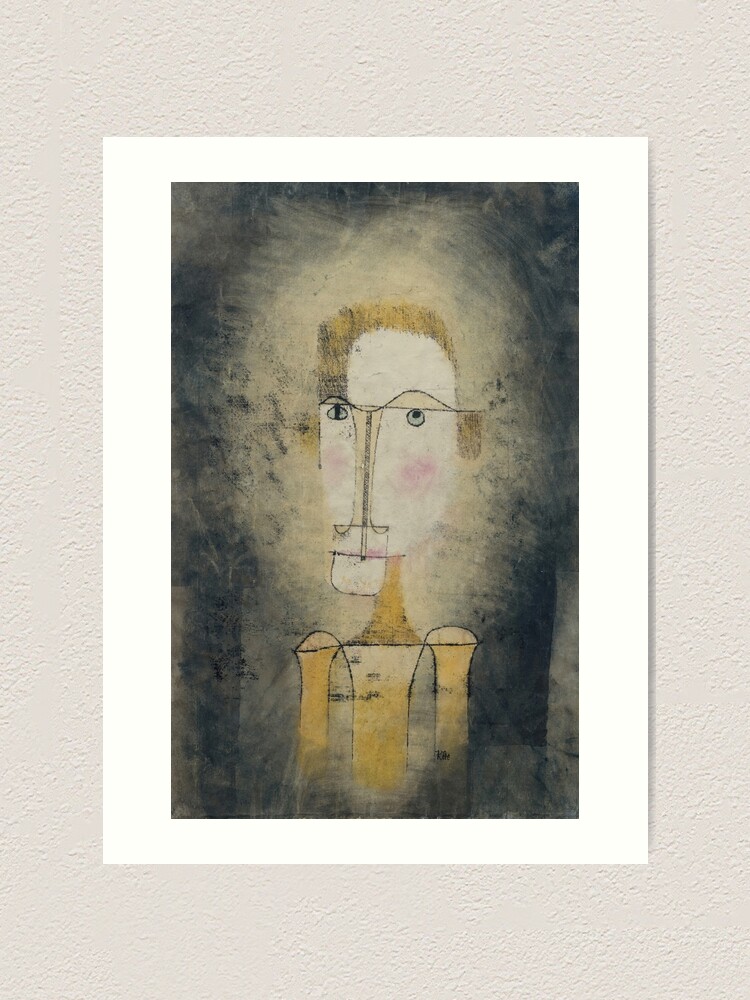The image features an abstract painting hung on an off-white, textured wall resembling deep spackle. The painting, which has a white border—quarter-inch at the top and bottom, half-inch on the sides—is about 4 inches wide and 5 to 6 inches in height, making it rectangular. The primary subject is a surreal figure depicted in a style reminiscent of Picasso. The figure, rendered in desaturated yellow, features a long, oval-shaped white face adorned with a heavy blush and peculiar eyes—one being an oval with a blue sclera and a black stripe, the other round with a round pupil. A curved unibrow arcs across the face, dipping at the bridge of the nose and rising again, while the nose itself appears like a long zipper. The expression is completed with a flat, thin-lipped mouth and a wide U-shaped chin. The background of the figure transitions from dark gray at the periphery to a tan color, smudged into the surrounding black. The entire composition is framed against the eggshell white wall, creating a striking contrast with the abstract, color-rich subject.